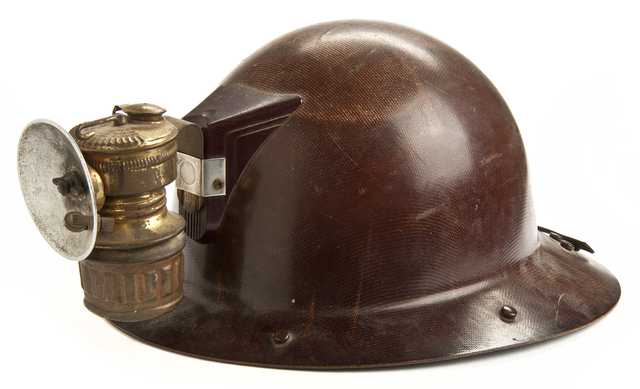The image depicts a vintage coal miner's hat made of a dark brown, metallic material with a shiny, yet worn and tarnished surface, showing scuff marks and a dent on the side. The hat is round with a brim adorned with rivets, displaying a mix of silver and brass accents. A notable feature of the hat is the attached canister-style headlight, which includes a bell-shaped component likely meant for holding fuel to keep the light burning. The headlight, built from brass and silver, would have been used by miners to illuminate their path while working underground. The background of the image is white, making the detailed wear and tear of the helmet, indicative of frequent use, prominently visible. The hat is positioned at an angle, emphasizing its rugged and historic nature.